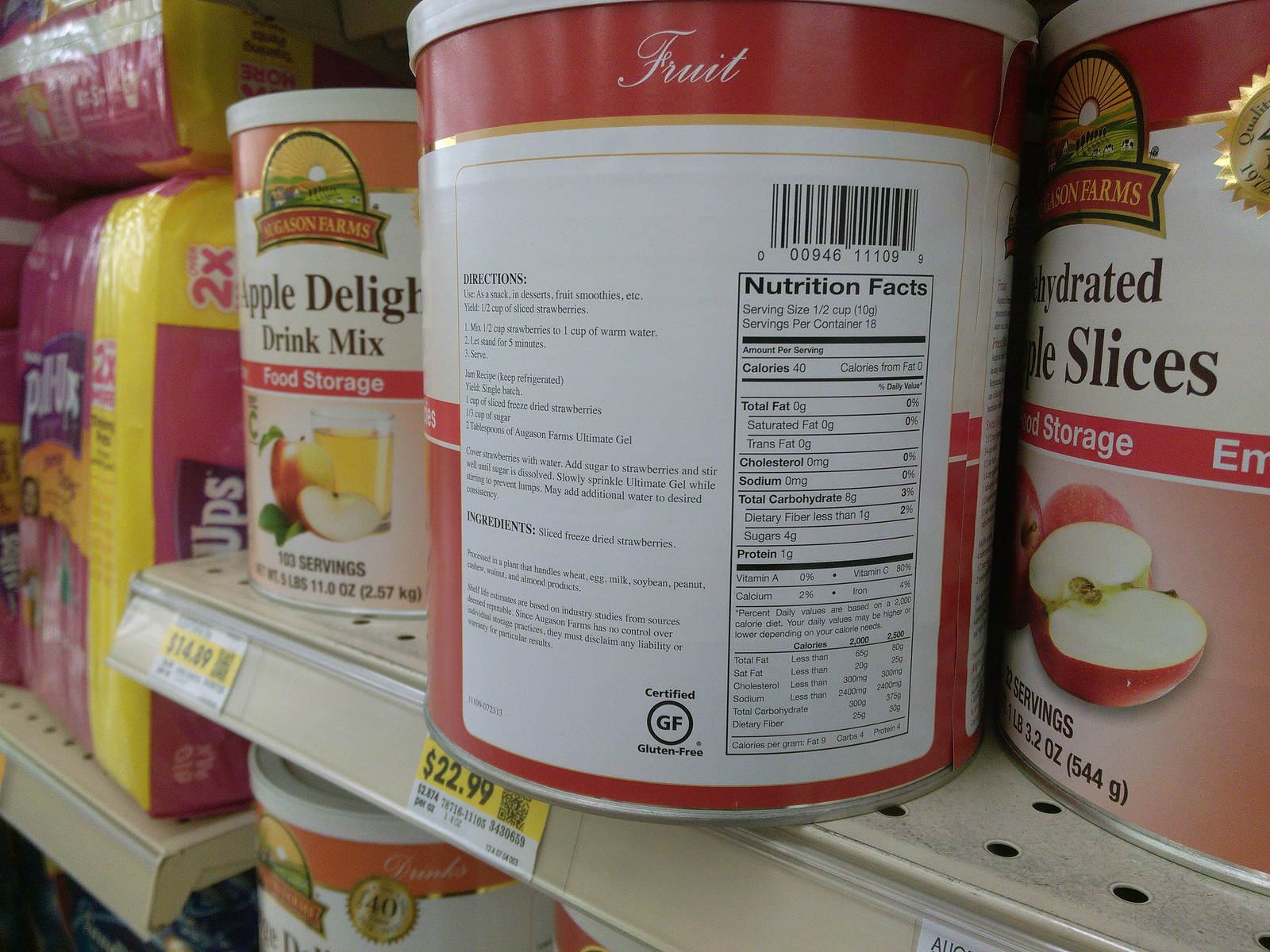This detailed colour photograph captures a close-up of products displayed on pale, creamy metal shelves, perforated with small black holes. Prominently featured are large canisters taking up about four-fifths of the image's height. The canisters, primarily from a brand named "Something Farms," include "Apple Delight Drink Mix" and "Dehydrated Apple Slices." The "Apple Delight Drink Mix" canister displays a picture of an apple in a clear glass and is labeled with nutritional information and a gold emblem, although the brand name is partially obscured. The "Dehydrated Apple Slices" canister features imagery of sliced apples and has a prominent red and yellow rim. The prices for these products, visible on stickers featuring an upper yellow section and a lower white section with black text, are $14.89 for the drink mix and £22.99 for the dehydrated apple slices.

On the left side of the shelf, there are packages of children's pull-ups or diapers. These packages are pink with yellow edges and display a little girl on the front, along with the size indication "2X." The use of bright colors and clear labeling makes the products easily distinguishable in the retail environment, enhancing their visibility and appeal to shoppers.